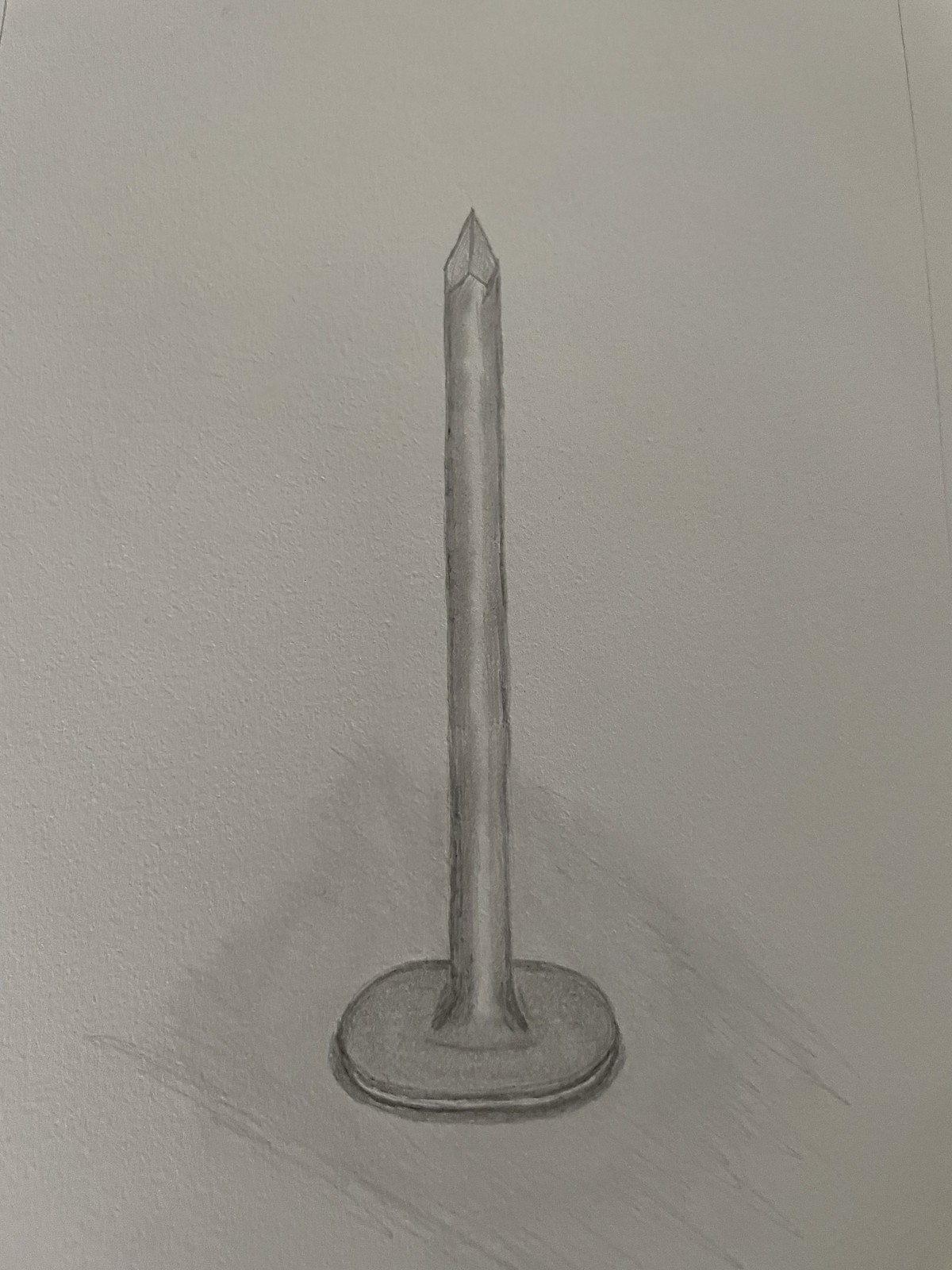This photograph showcases an exquisitely detailed pencil drawing of a nail, rendered with remarkable precision using graphite pencils on textured white paper. The head of the nail, meticulously shaded and round in shape, is positioned on the surface, allowing the nail to stand vertically with its sharp point directed upward. The intricate shading and delicate lines capture the light and shadow with astonishing accuracy, emphasizing the angles converging to form the sharp tip of the nail. The artist's skillful use of graphite conveys the metallic texture and reflective quality of the nail, creating a stunningly realistic and lifelike representation.